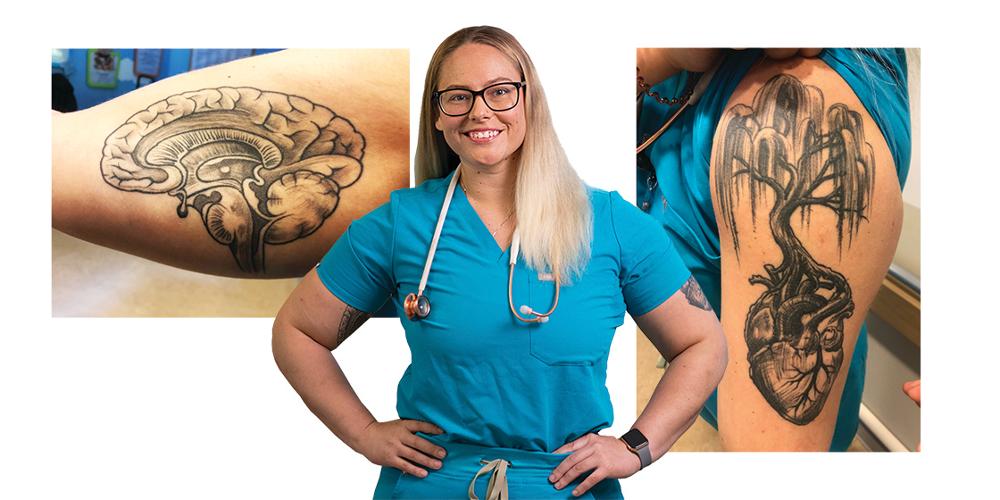The image is a detailed collage centered around a cheerful woman who appears to be a nurse or doctor. She stands confidently with her hands on her hips, smiling broadly with her teeth showing. The woman is Caucasian with straight blonde hair that has highlights towards the bottom, and she wears black glasses. She is dressed in blue scrubs and has a white stethoscope around her neck, as well as a smartwatch on her wrist. Flanking her central image are close-up shots of her tattoos, which are black and intricate. On the left, there's a side-view tattoo of a human brain, while on the right, there's a tattoo of a human heart with veins artistically forming a tree that resembles a willow tree. The background of the collage is plain white, emphasizing the details of the woman and her tattoos.